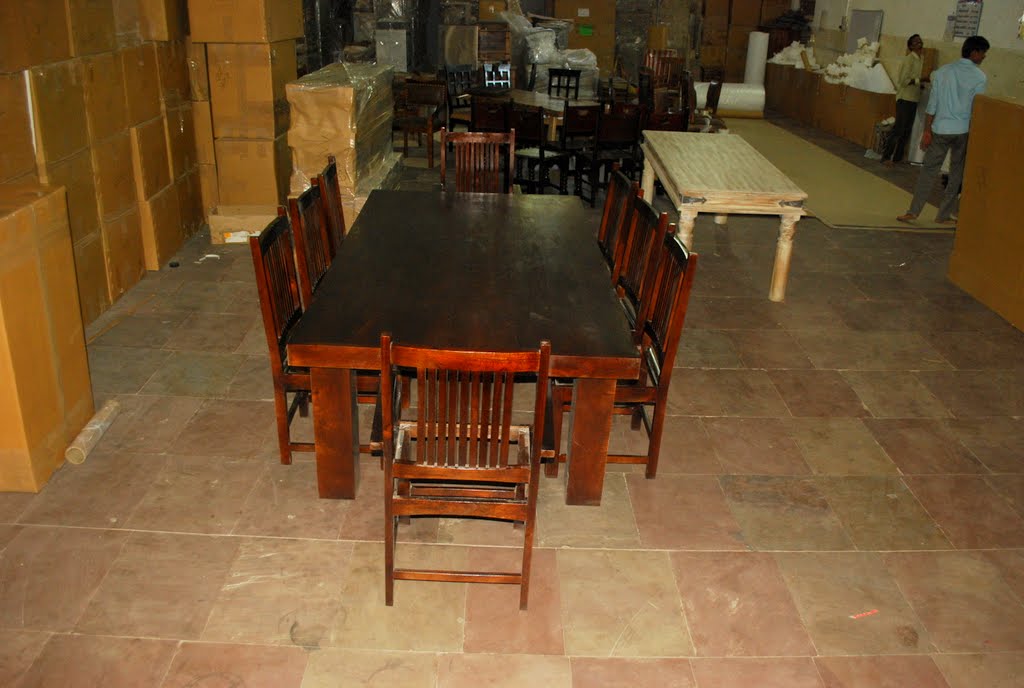The image shows the interior of what appears to be a warehouse or furniture store. In the left foreground, there's a large stack of different-sized cardboard boxes sealed with brown parcel tape. Dominating the foreground is a dark oak dining table with a rich mahogany color, cherry red tint, and eight matching wooden chairs arranged around it—three on each side and one at each end. The chair closest to the camera is missing its seat cushion, revealing a gap. The flooring consists of varied colored tiles, including salmon, yellowish beige, and some darker patches.

Behind this table at an angle, there’s another dining table made of lighter brown wood with six chairs featuring crisscrossed backs. Further back, another smaller table without chairs is visible. In the large room, other items of furniture are scattered around, lending an impression of a functional warehouse space. On the right side of the image, two men are present—one facing away and the other to the right. In front of one of the men, there appears to be an olive-colored carpet or some cardboard material rolled out on the floor, as though they are preparing the room for something or packing an item.